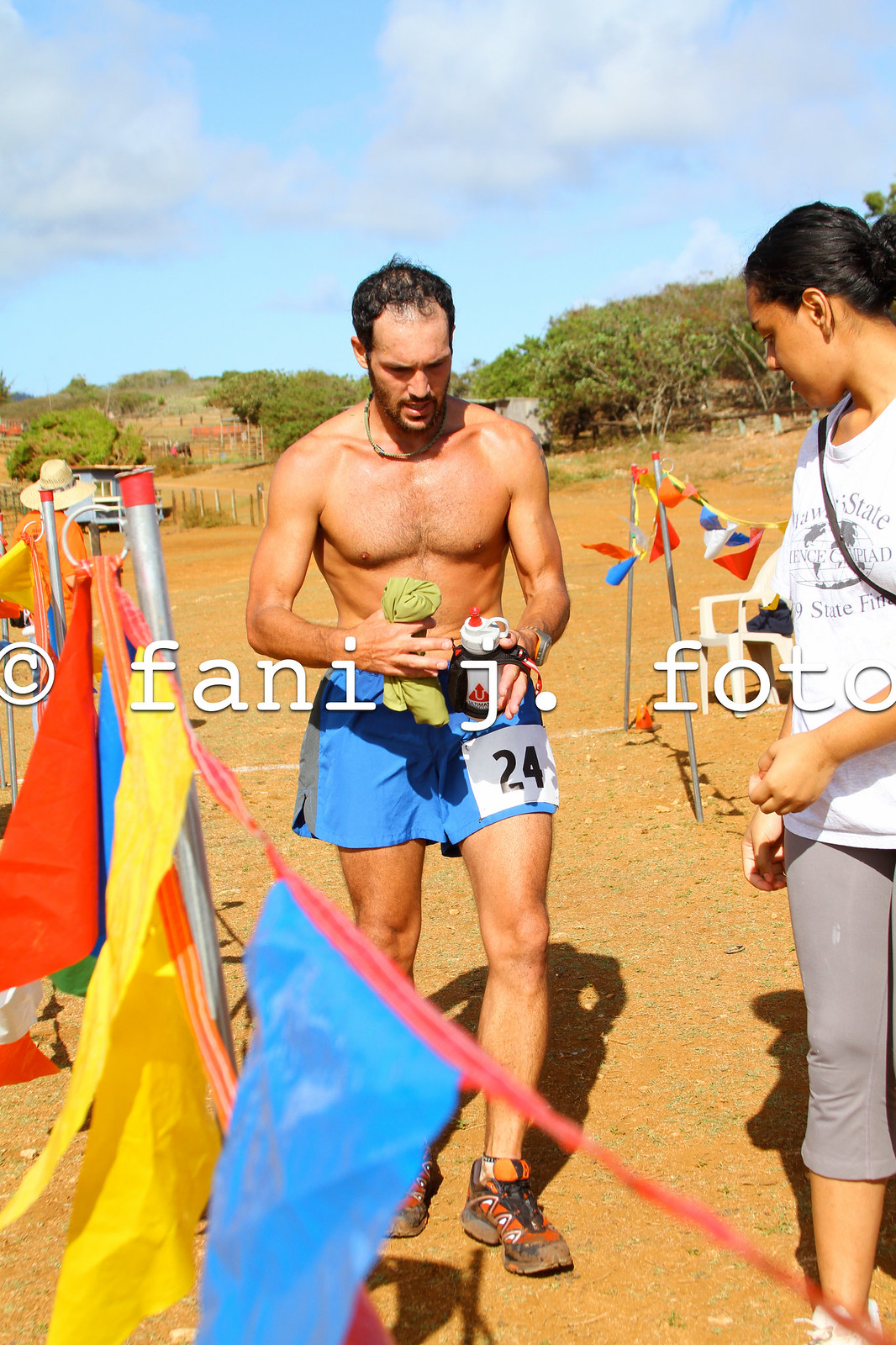In this horizontal rectangle-shaped photo, two people are outdoors during the day. Dominating the center is a fit, shirtless man, who has tan skin and black, slightly receding curly hair, resembling a lean Jeremy Piven. He sports blue running shorts, branded with a white square and the number '24' on his left leg, and has cross-trainer shoes on. Around his neck is a band-style necklace. In his right hand, he holds a green cloth, likely his t-shirt, and in his left, a white can which might be water or an energy drink. His posture and attire strongly suggest he is participating in a race or an intense workout.

To the right, a woman with black hair styled in a bun, dressed in a white t-shirt and gray cropped leggings, appears to assist him, possibly handing over necessary items. She carries a crossbody sling. The ground beneath them is light brown, resembling a mix of dirt and gravel, typical of a rugged nature trail.

In the background, under a blue sky sporadically decorated with fluffy white clouds, are some trees and small village-like buildings, adding depth to the scene. An individual wearing a hat is also faintly visible amidst the trees. Flanking the scene on the left side of the photograph, a line of small, colorful triangular flags—blue, yellow, and orange—hang from strings attached to poles, defining the race area. The photo bears a watermark, "FANIJ.FOTO," in white text.